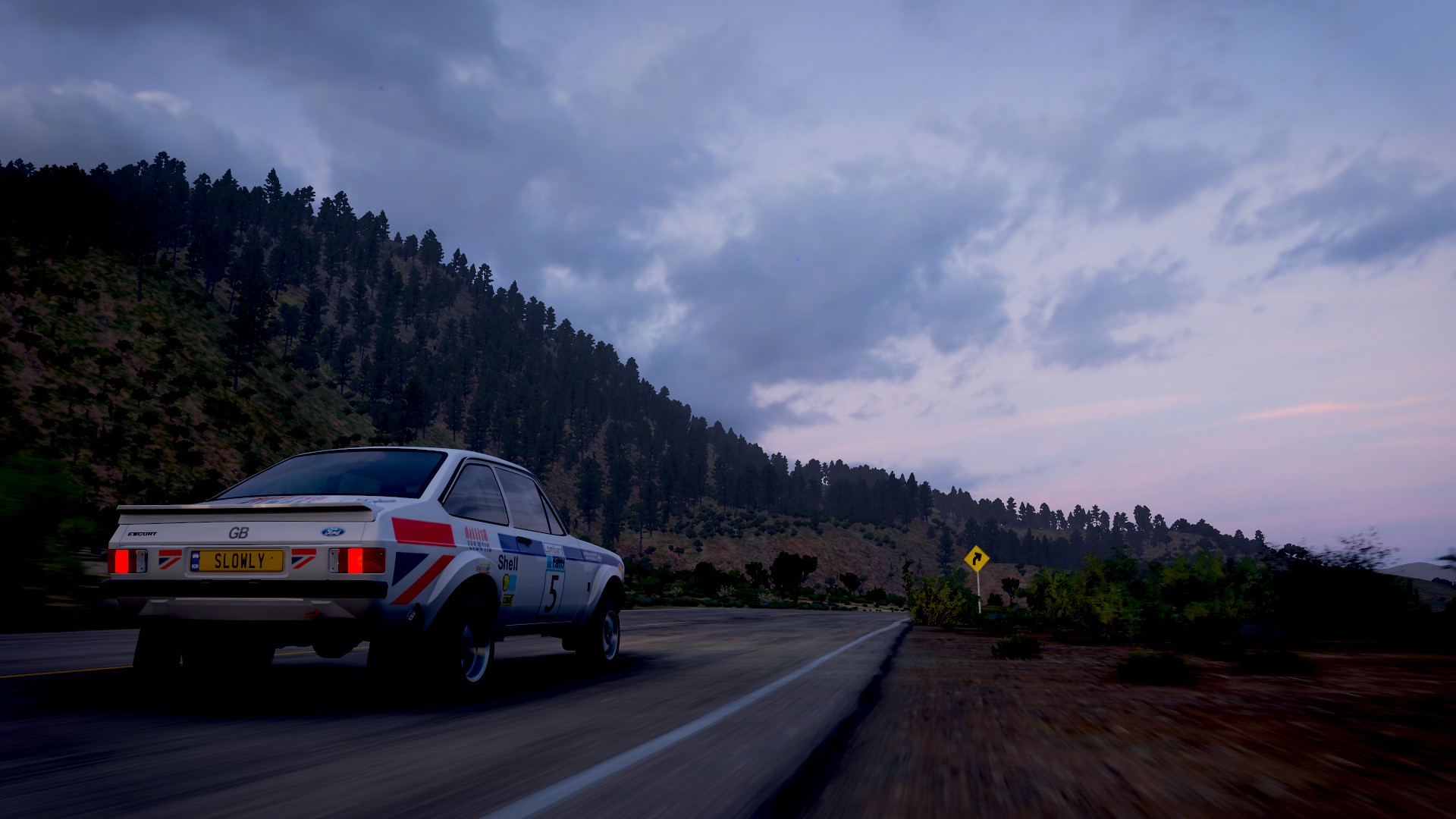This photograph captures a dramatic evening scene of a solitary race car navigating a tree-lined countryside road. The setting sun casts a dusky glow over the landscape, with the darker, partly cloudy sky tinged with hints of pink. The road curves ahead, indicated by a yellow street sign with a right-hand arrow. A white car with blue and red stripes dominates the scene, its large racing tires gripping the asphalt. Emblazoned with rally insignia, including the number 5 on the door and logos like Shell Oil, GB, and Ford on the back, the car sports a distinctive fin and a yellow license plate that reads "Slowly." The illuminated headlights pierce the dimming light, adding drama to the scene as the car approaches a bend in the road. Majestic trees dot the mountainside on both sides of the road, complemented by smaller bushes, which complete the picturesque, rural setting. The solitary nature of the drive suggests a moment of intense focus, with the race car adventuring through this serene but challenging terrain.